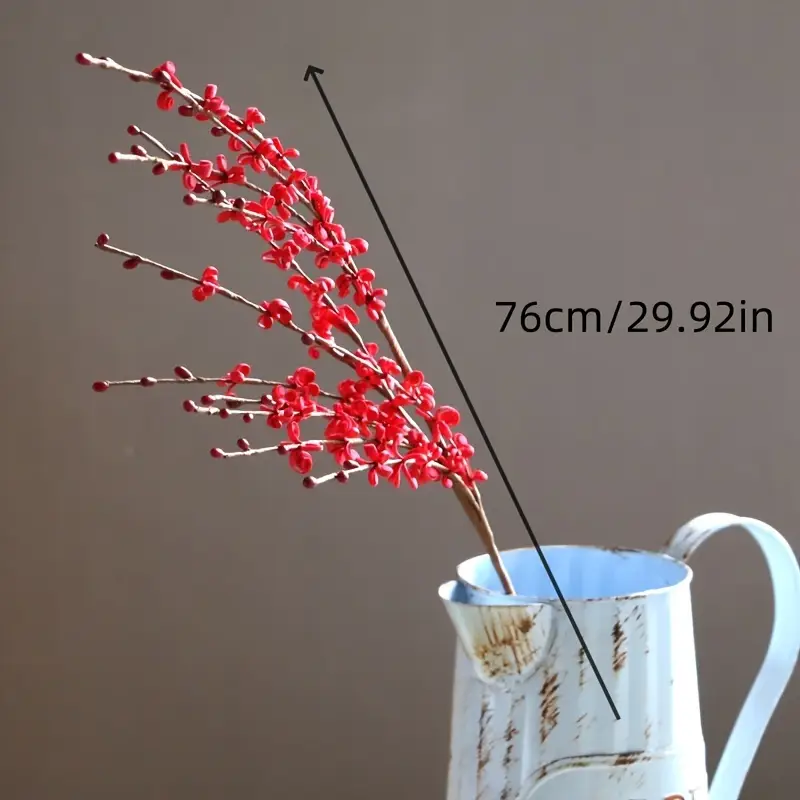The image depicts a white, metal pitcher with scratch-like brown markings that resemble rust. Sticking out from the pitcher is a single thin branch with multiple offshoots, each adorned with small, dark red flower buds. The branch, which is measured with a diagonal black arrow to indicate its length of 76 centimeters (29.92 inches), contrasts against an ombre brown background that is lighter on the right and darker on the left. The lighting highlights the right side of the scene.